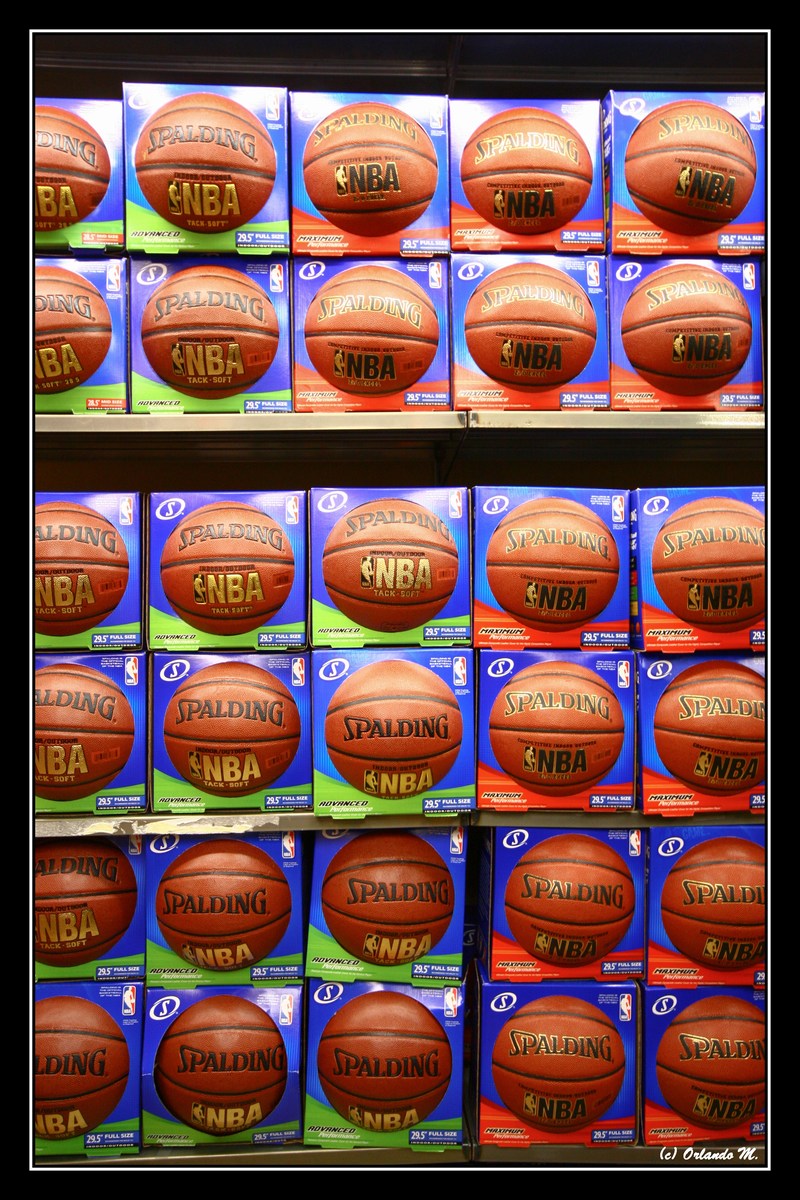This detailed indoor color photograph resembles a postal card with its distinct white border and the signature "Orlando M ©" in the lower right corner. The image showcases a neatly arranged display of brand new Spalding NBA basketballs, each in square cardboard boxes with the ball protruding through the front. The basketballs vary in branding and design: some feature gold NBA lettering with black Spalding logos, while others have black NBA lettering with black Spalding logos. Additionally, some boxes include green or red stripes at the bottom. The basketballs are organized meticulously into five columns and six rows, creating a visually appealing grid. The identification text on each box is too small to be legible, and the light reflects off the boxes, indicating their pristine condition.